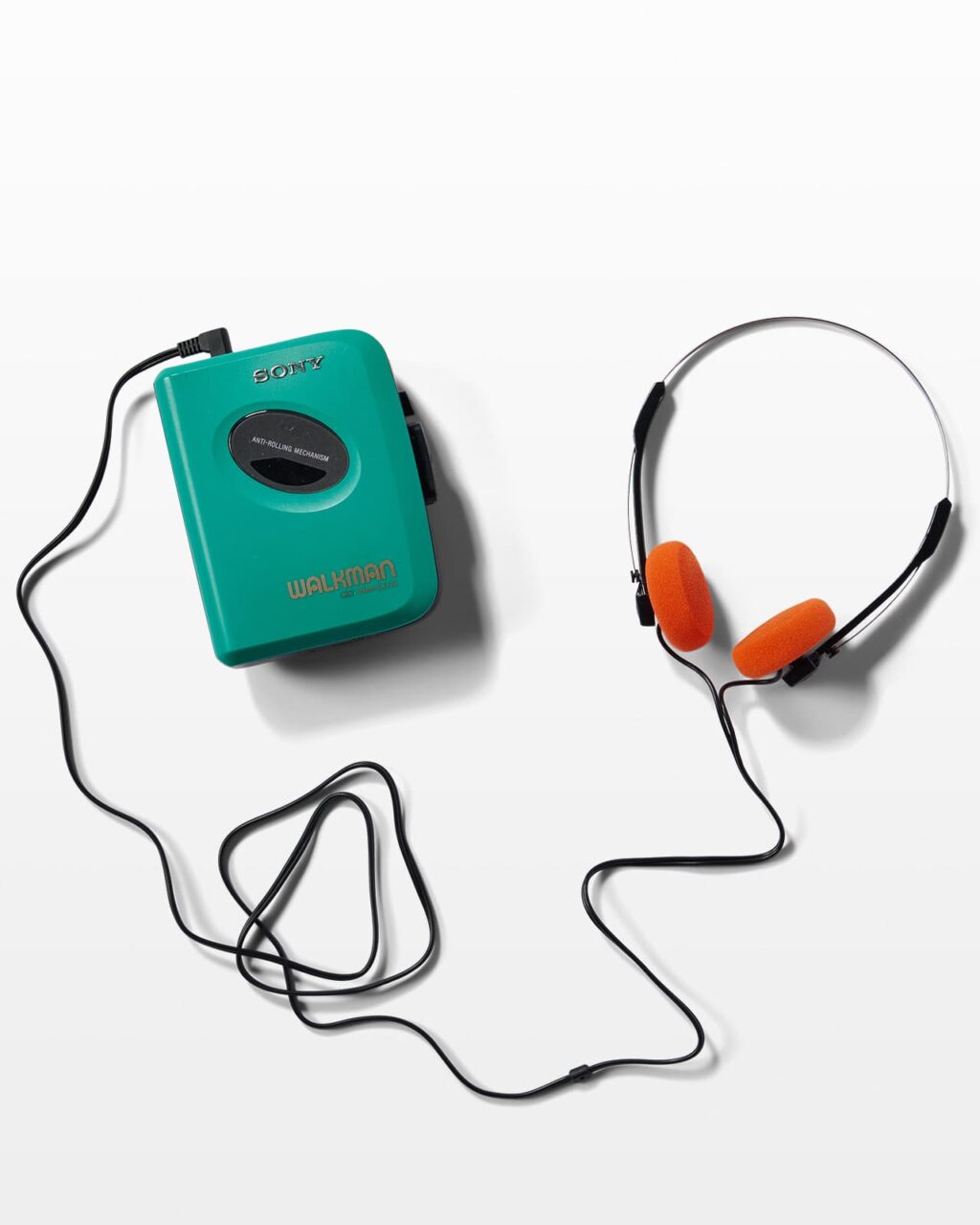This photograph features a vintage Sony Walkman displayed on a pristine white background. The Walkman boasts a blue-greenish hue and prominently displays "Sony" in silver lettering at the top and "Walkman" in gold lettering at the bottom. In the center of the device, an off-center oval label reads "anti-rolling mechanism." On the right side, there are two black buttons, while a headphone jack emerges from the top left, with the black headphone cord looping over itself a couple of times before extending to the right side of the image. The headphones attached to this Walkman have bright orange earpieces and black sides, connected by a slender silver wire that curves over the head. This combination of features suggests it might be an early model or a modern remake of the classic Walkman.